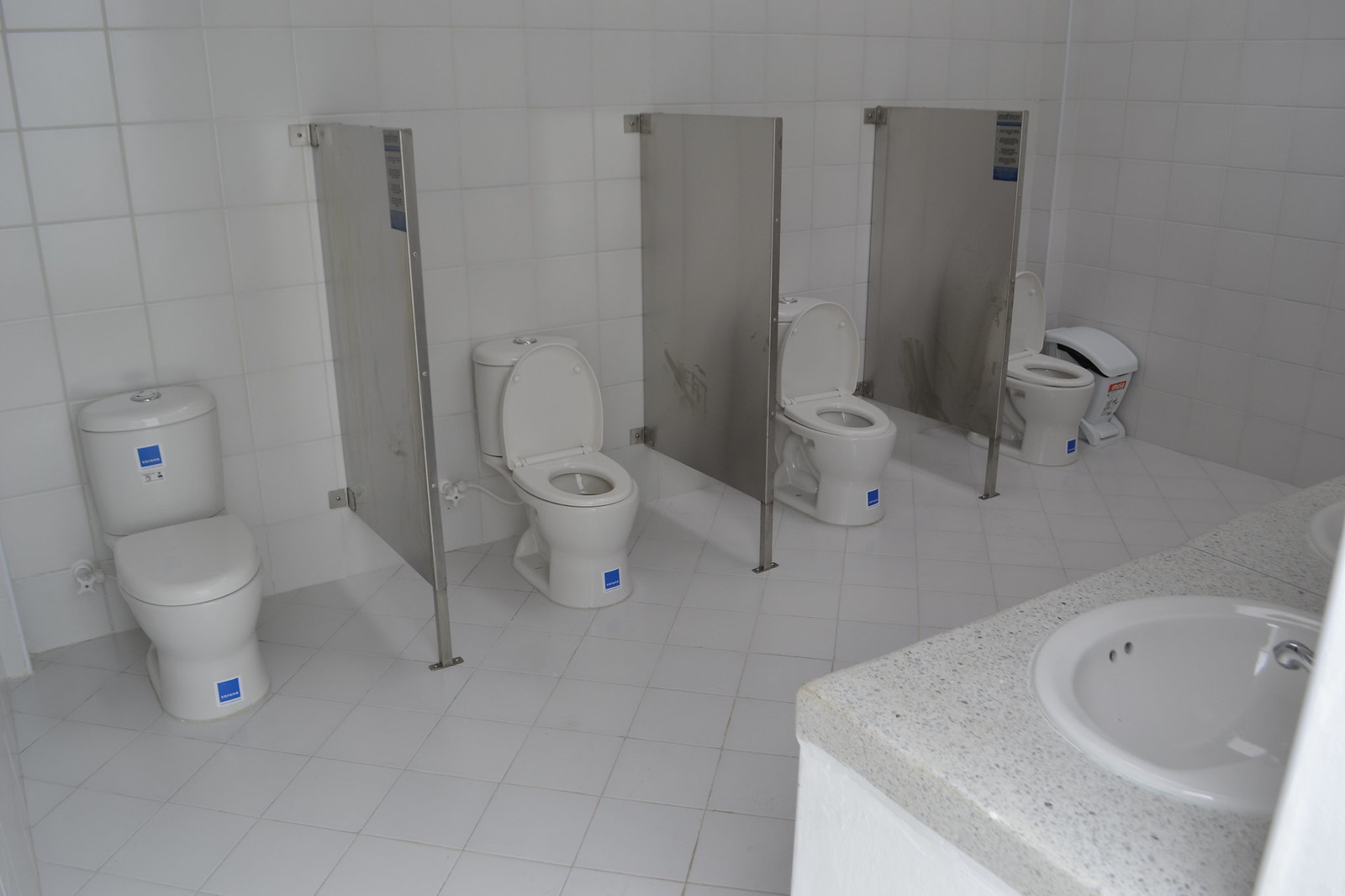This photograph showcases a possibly dormitory or public bathroom with a slightly unsettling design. The space features four white toilets aligned against a wall adorned with white horizontal square tiles. Each toilet is separated by dark grey dividers, which appear to be made of possibly dark grey glass or steel sheets. The toilets are marked with blue stickers on both the toilet stands and cisterns, adding a touch of color to the otherwise monotonous white palette.

One distinct feature in this setup is the toilet on the far left, which has a closed seat lid, unlike the others, where the lids are open. To the right of the image, next to the rightmost toilet, stands a plastic white garbage can with a red label, resting against the tiled wall. Adjacent to this is a granite-effect countertop featuring a white basin and a corresponding white cupboard.

The flooring of the bathroom contrasts the wall tiles by featuring white tiles arranged in a diamond layout, producing a visually distinct pattern. Additionally, in the foreground and extending further along the wall, there is a countertop in a Corian-like design, housing a sink with a silver tap and decorative black-speckled cream surface, hinting at more sinks in a possible row beyond the frame of the photo.